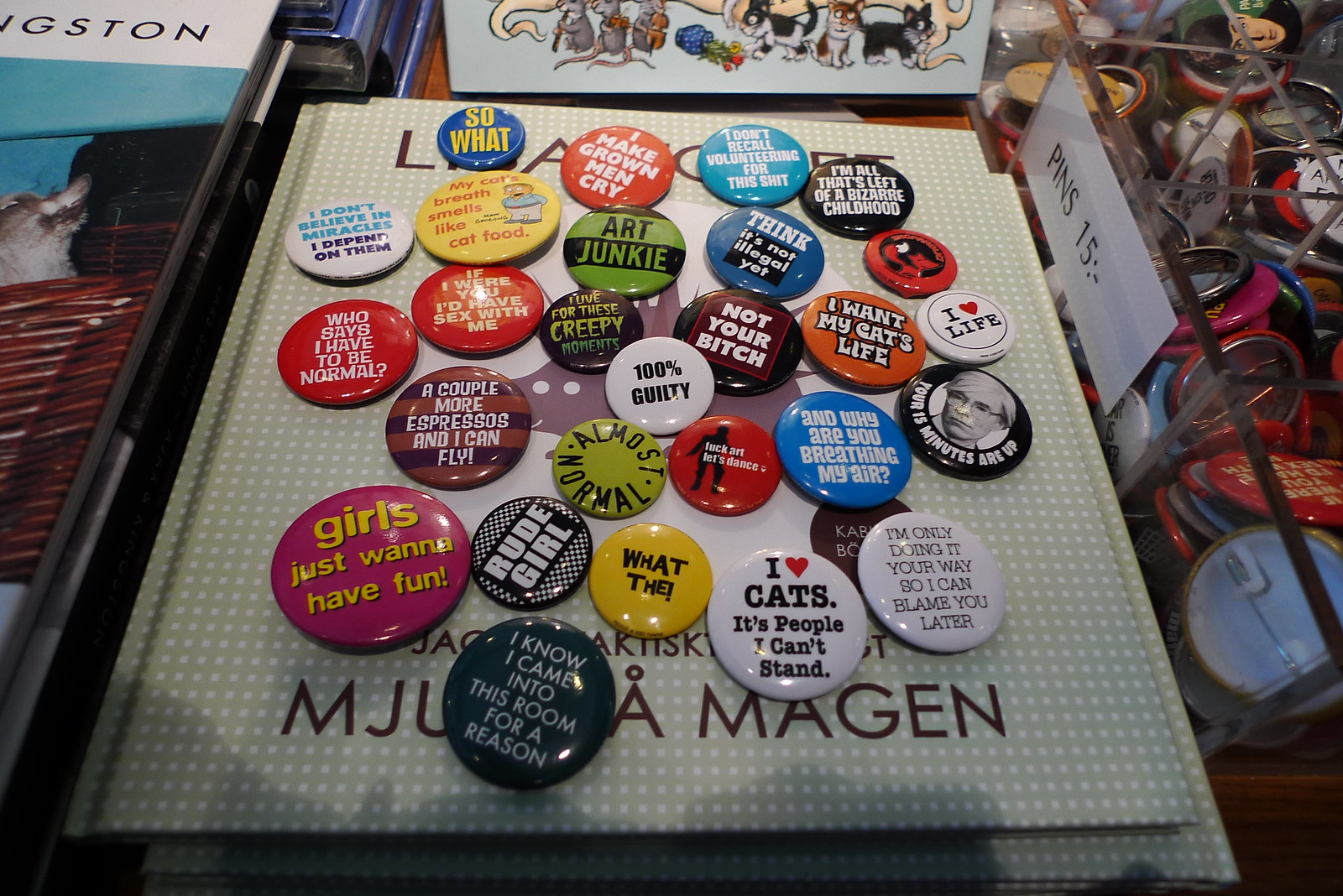The photograph, seemingly taken indoors, showcases a vibrant collection of pin-on buttons meticulously arranged on a flat, light green and white checkered book, the partial title visible as "M-J-U," "A," and "M-A-G-E-N." These buttons feature a variety of bold and provocative statements, including "So what?", "I make grown men cry," "Art junkie," "Not your bitch," "100% guilty," "Fuck art, let's dance," and "I heart life." Other notable pins include "I'm only doing it your way so I can blame you later," "Girls Just Wanna Have Fun," "Rude Girl," "I Heart Cats. It's People's Lives I Can't Stand," and the lengthy "If I Were Something To You I'd Have Sex Every Day With You." The pins are accompanied by another identical book beneath and a stack of books to the left with indiscernible titles. To the right, transparent plastic cubes labeled with "Pins 15" contain additional buttons, suggesting these items might be for sale. In the background, a book featuring cartoon animals, possibly rats and cats, is partially visible, adding an intriguing, whimsical element to the overall scene.